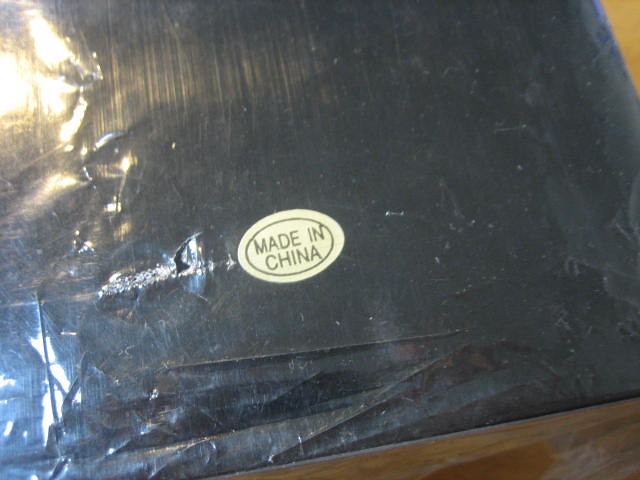The photograph captures a close-up, detailed view of a small section of a slightly worn wooden tabletop, visible in the bottom and upper right-hand corners. Dominating the image is a square object with a black, slightly reflective, plastic-covered surface. The plastic, which appears somewhat crumpled and even torn in one spot in the upper left-hand corner, has a slight glare from reflected light. Attached to this black surface is a small, oval-shaped gold sticker bordered by a thin black line. Inside the black border, in clear black print, is the text "Made in China." The extreme zoom on the object obscures its full identity, leaving only the black square and its plastic cover discernible.